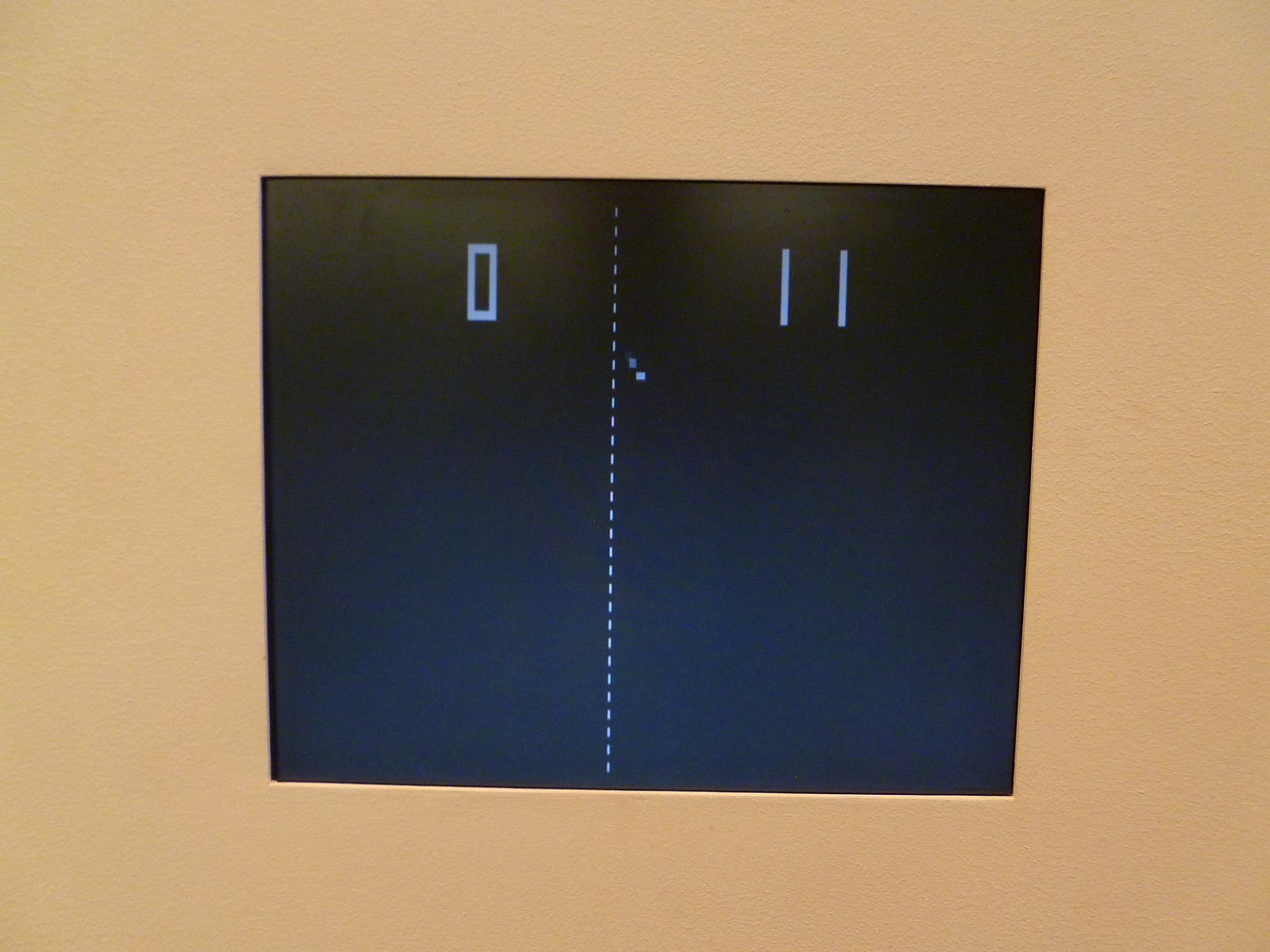This photograph features a central black square screen, which is bordered by a thick, cream-colored margin. Dividing the black screen down the middle is a vertical white dotted line. On the left side of this line, there is a white "0," and on the right side, there is a white "11." A white, cursor-like symbol is positioned near the dotted line, adding an element of focus to the minimalistic display. The substantial white border around the central black screen creates significant negative space, emphasizing the minimalist design. The overall appearance is reminiscent of vintage computer interfaces or early video game graphics like Pong, although it retains a distinct simplicity and mystery.